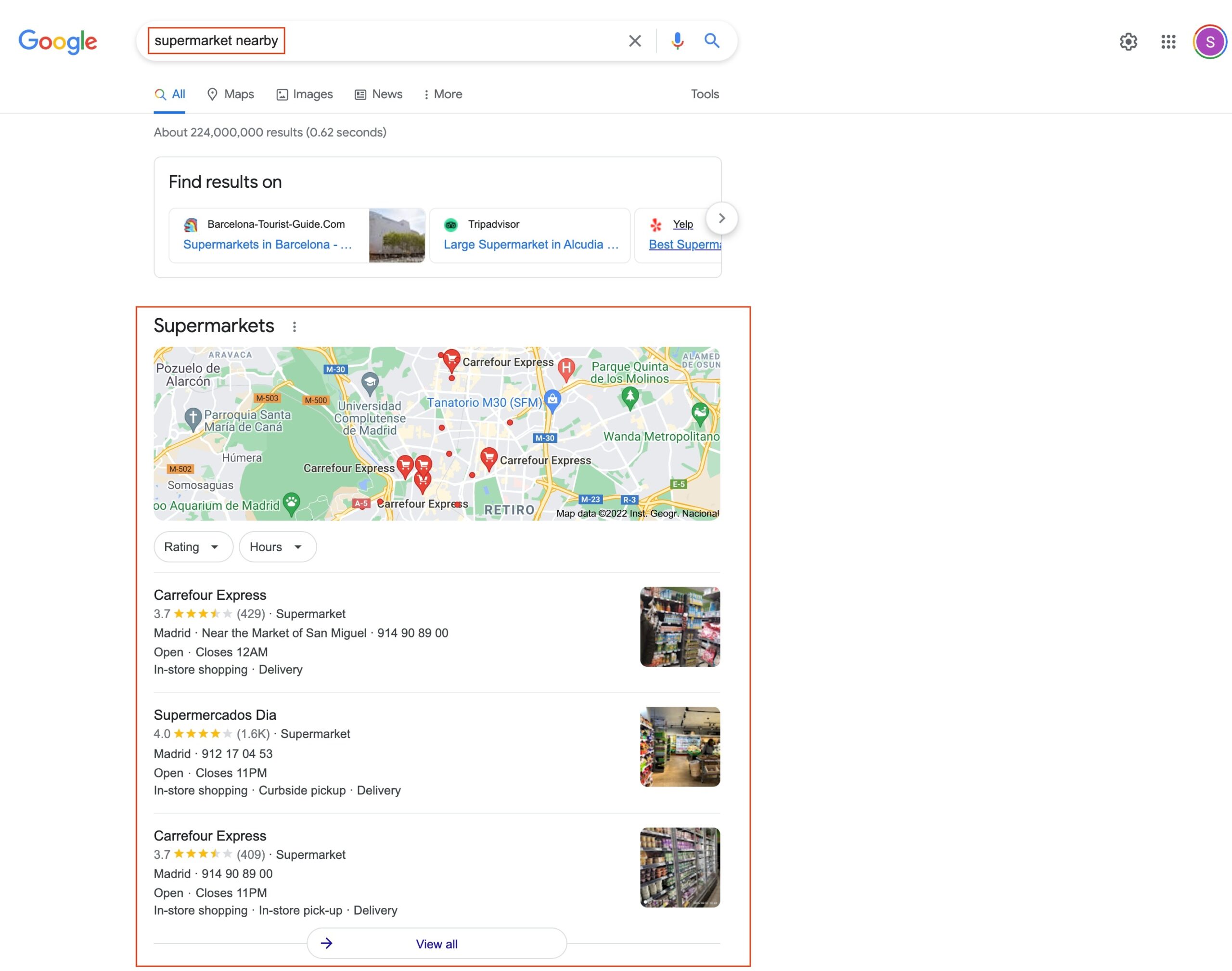This vertical image depicts a screenshot of a Google search results page on a white background, as viewed on a computer or smart device. In the top-left corner, the Google logo is displayed prominently in its iconic blue, red, yellow, blue, green, and red colors. To the right of the logo, a search bar is visible with the query "supermarket nearby" highlighted by a red rectangle. The search bar contains the gray "X" to clear the text, a microphone icon for voice input, and a magnifying glass icon for initiating the search.

Directly below the search bar, towards the left, the "All" tab is underlined in blue, indicating it is the active tab. To the right of "All," additional tabs are available: Maps, Images, News, and More. Farther to the right is the "Tools" option. Scanning back up to the top-right corner, icons for settings, Google apps, and a user profile denoted by an "S" inside a circle are displayed.

Returning to the main content area, on the left side, the number of search results and the time taken to generate them are noted. Prominent websites listed among the search results include barcelonatouristguide.com, TripAdvisor, and Yelp. A map highlighting nearby supermarkets is also visible, showcasing specific options such as Carrefour Express and Supermercado Sedia. Each supermarket result includes a rating (indicated by stars), the number of reviews, the address, phone number, operating hours, and a thumbnail image next to each listing.